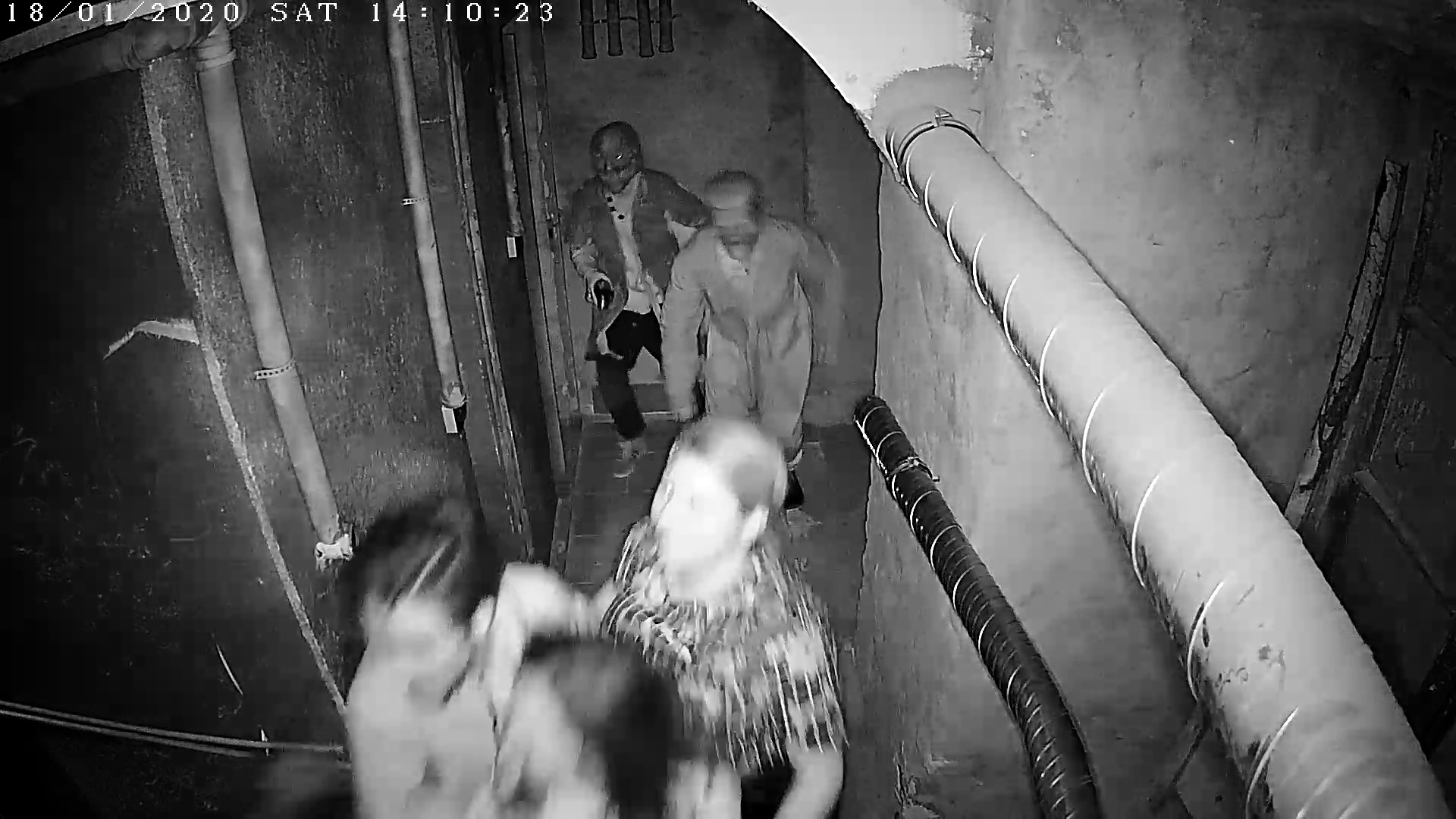This black and white photo, seemingly captured by a security camera on January 18th, 2020, at 14:10:23, depicts a chaotic scene in a basement-like stone corridor. The timestamp is visible in the top left corner. The image shows five blurry figures, likely due to their rapid movement, suggesting they are in a hurry or running. The person in the far back appears to be wearing dark pants and a light shirt under a jacket and may have a mask on, adding a sense of mystery or fear. Beside them, another individual is distinguishable by a hat and a jumpsuit. The three people in front are extremely blurry, reinforcing the sense of urgency. The corridor is lined with pipes, with two running horizontally on the right side and two vertically on the left, further suggesting a basement or industrial setting. The photo exudes an eerie, haunted atmosphere, possibly indicating a scene from a haunted house attraction or a similar event.